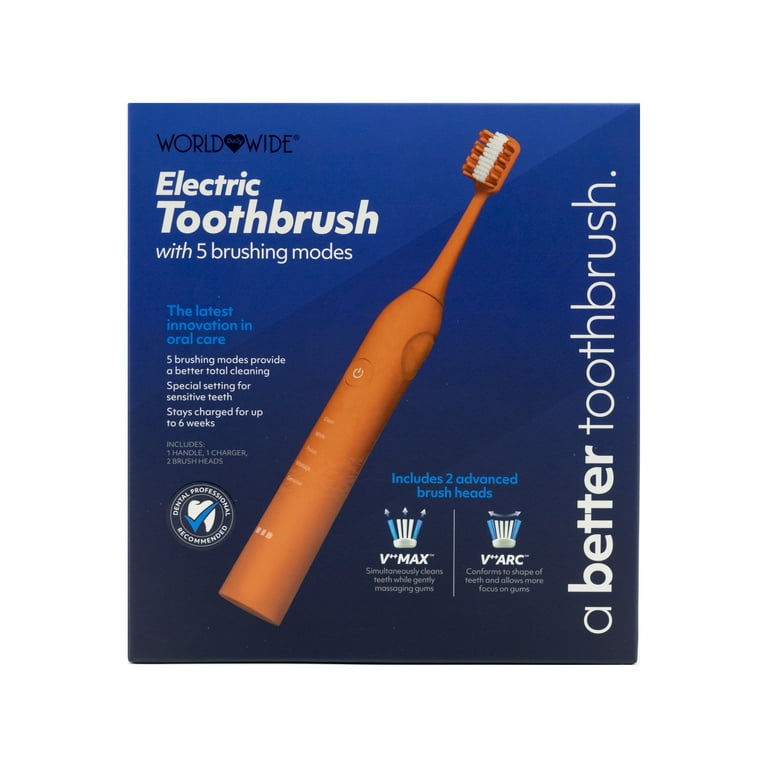The advertisement showcases a prominently featured orange electric toothbrush positioned diagonally in the center against a dark blue background. The toothbrush has a large, thick handle with a white power button, likely an LED, and a white stripe running through the middle of its orange bristles. The text at the top left reads "Worldwide," possibly the brand name, followed by "Electric toothbrush with five brushing modes" in bold white letters. Below that, blue text highlights "The latest innovation in oral care." A smaller white text further elaborates on the modes, including a special setting for sensitive teeth and a six-week battery life. It mentions the package includes one handle, one charger, and two advanced brush heads—the V-Max and the V-Arc. Positioned vertically on the right side, the caption "A Better Toothbrush," with "Better" in bold, emphasizes the product's superior quality. Additionally, an image of a tooth with a checkmark and the note "dental professional recommended" adds credibility to the advertisement.